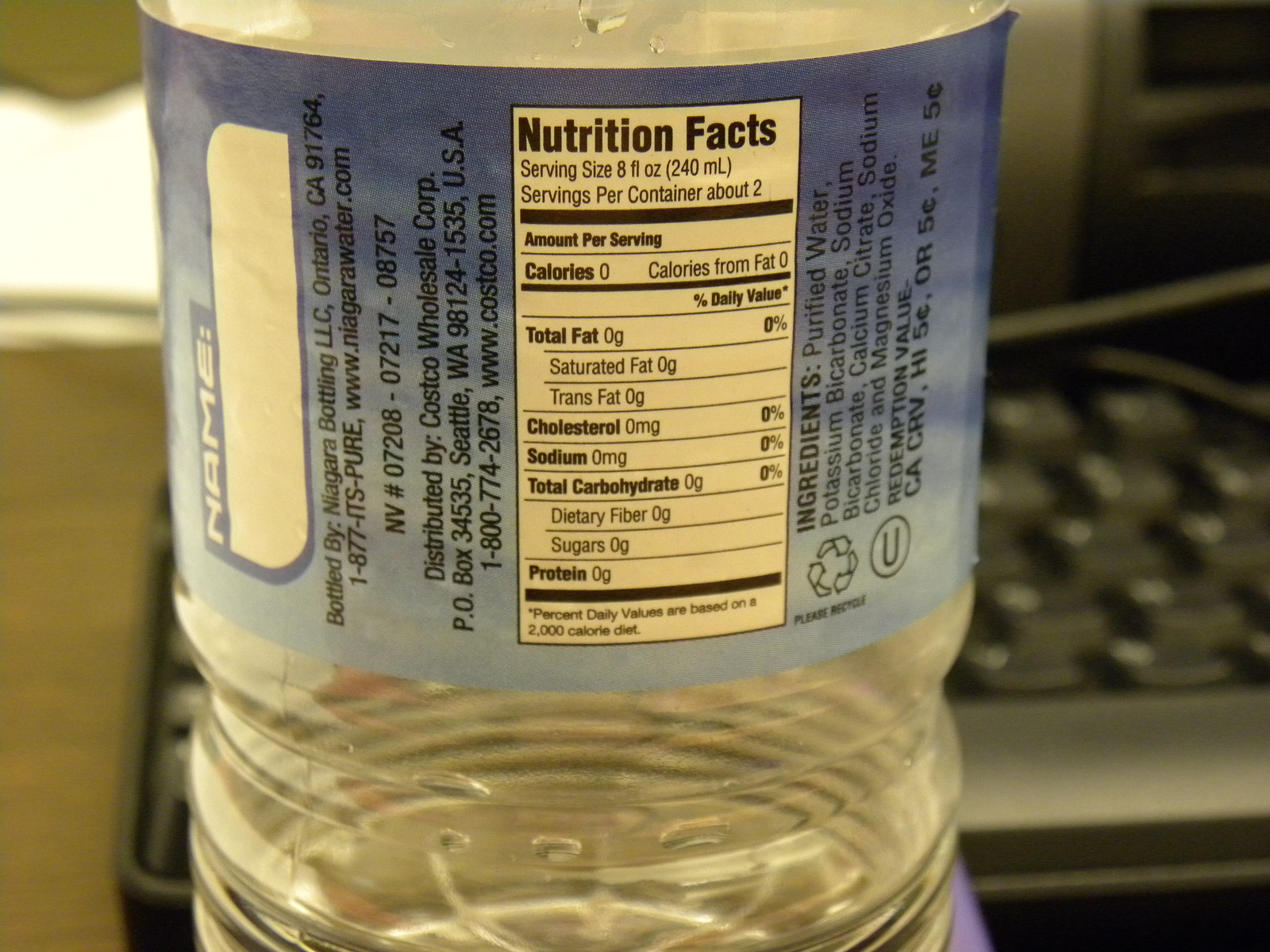In this horizontal rectangular photograph, the central focus is a close-up of a transparent plastic water bottle, prominently positioned vertically in the middle of the frame. This bottle is bottled by Niagara Bottling LLC, located in Ontario, CA 91764, as detailed in black text on the bottle's blue label. The label, which spans from just below the bottle's top to about two-thirds of its height, prominently features a white rectangle containing the nutrition facts, presented in black text. The serving size is listed as 8 FL OZ (240 ml), with about 2 servings per container, and the nutrition details show nearly all components as zero.

Beside the nutrition information, additional text on the label lists the ingredients, which include purified water, potassium bicarbonate, sodium bicarbonate, calcium citrate, sodium chloride, and magnesium oxide. The label also mentions a phone number and a website for further information. The water bottle appears nearly empty, with just a few water droplets visible inside.

The background of the image is intentionally blurry, emphasizing the water bottle itself. It depicts a mix of beige and gray tones, potentially resembling a kitchen with stainless steel elements, or perhaps a workspace that includes a computer keyboard and other indistinct objects. Light is streaming in from a window in the upper left corner, adding a soft, natural illumination to the scene.